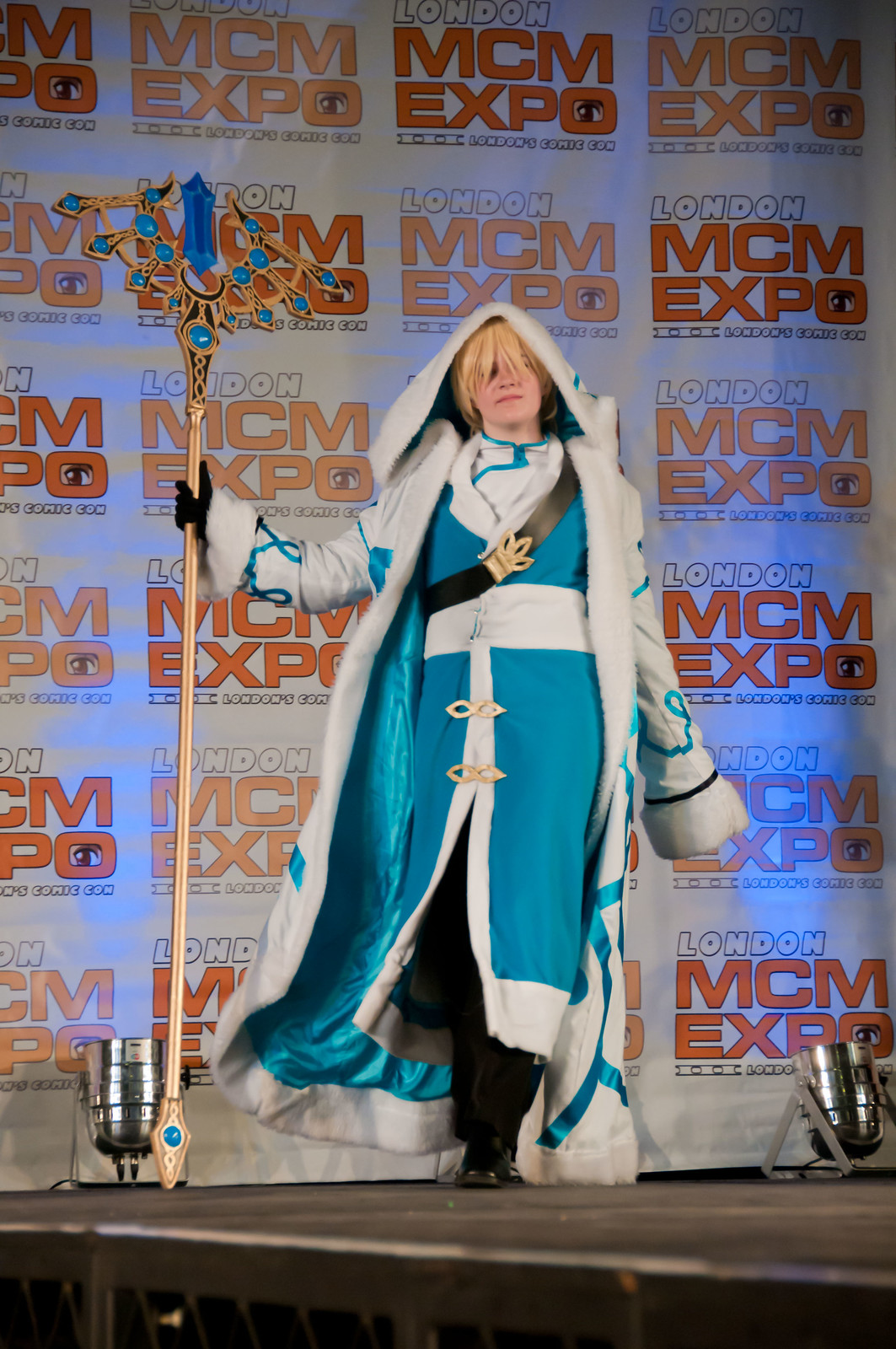This image captures a person, possibly a woman, walking on stage at the London MCM Expo, indicated by the repeating banners in the background that prominently display the "London MCM Expo" text in alternating white and orange colors. The person is donned in a striking blue and white ensemble that blends elements of medieval and magical attire. The costume features a flowing white and blue robe with large sleeves and a voluminous hood that drapes over their head, partially obscuring their straight blonde hair, which falls down to their nose. The ensemble is completed with puffy black gloves and black pants, with the inside of the robe lined in a shiny, velvety blue fabric. In their right hand, they hold an ornate golden staff adorned with blue jewels; the staff has a splayed design at the top, resembling peacock feathers, with a single jewel accentuating the bottom. The vibrant costume and prop suggest this may be a cosplay event where participants dress as characters from various fantastical genres.